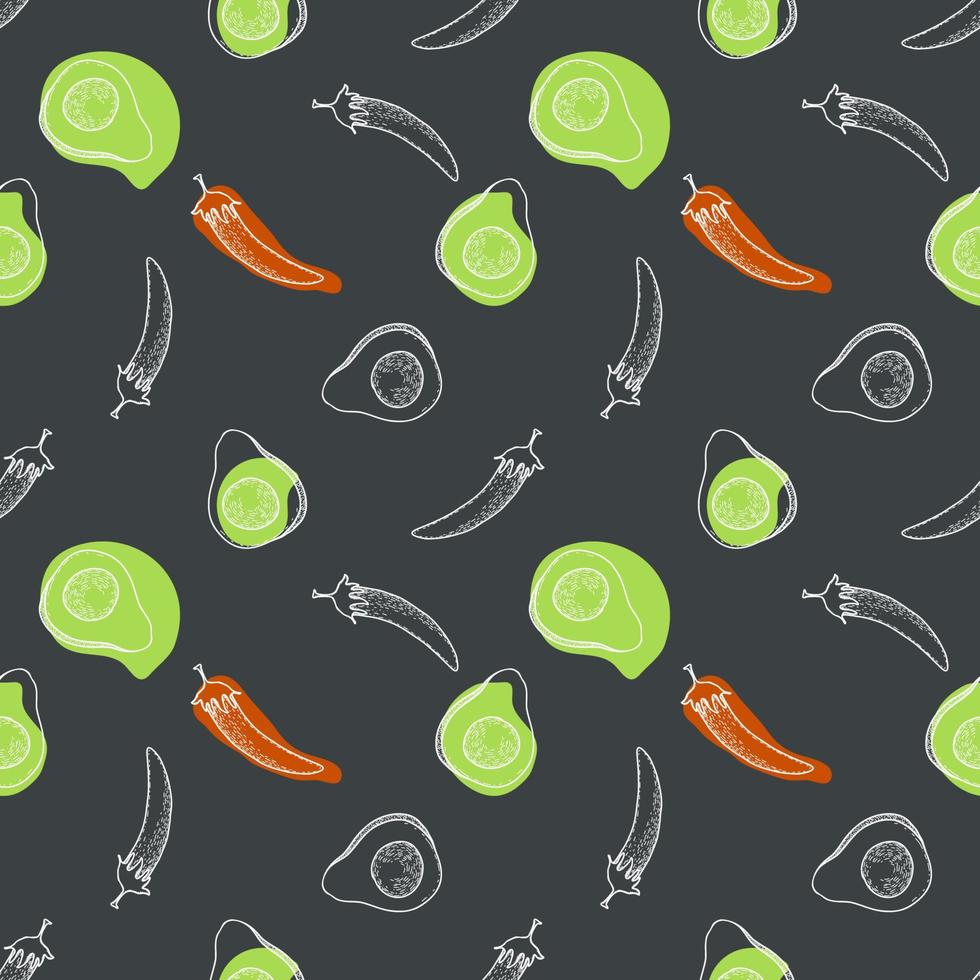This image features a dark gray background resembling a chalkboard or elegant wrapping paper. Diagonally arranged across the print are simple illustrations of avocados and peppers. The avocados are primarily green, though the coloring is imperfect, often straying outside the lines. The red peppers are interspersed in the pattern, with only a few colored in red—approximately one every three or four peppers. This vibrant pattern resembles a repeated sequence: avocado, red pepper, avocado, and so on. The overall visual effect is a mix of colored and outline illustrations, with some food items purely in white, contributing to a dynamic and artistic kitchen-themed design suitable for a cover of a cookbook, a placemat, or a kitchen towel.